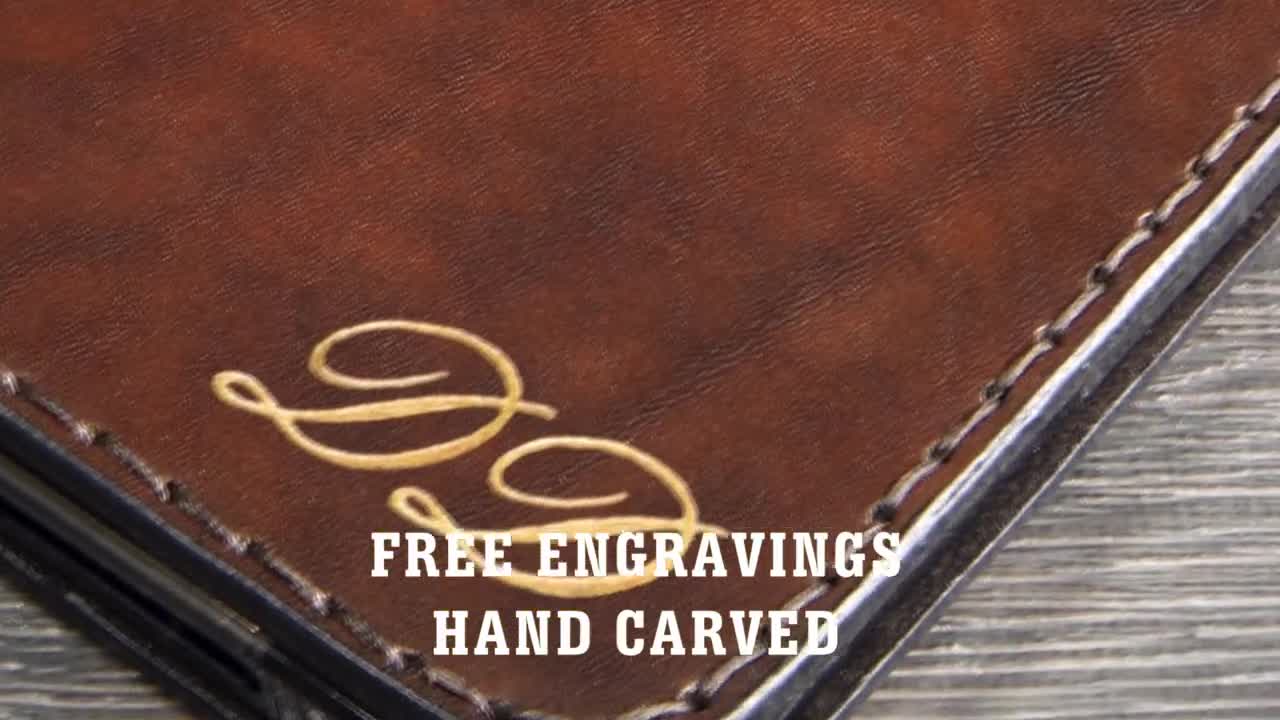The image depicts a color photograph of a brown leather object, potentially a notebook cover or wallet, characterized by its white stitching along the edges. This item, marked by the intricate details of genuine leather texture mingled with hints of black reminiscent of cowhide, shows two gold-etched D's on the bottom right corner. The inscription "free engravings, hand carved" is prominently displayed in white block letters across the bottom of the image. This brown leather item rests on a light gray wooden table, providing a contrasting backdrop that highlights the leather’s rich, dark tones.